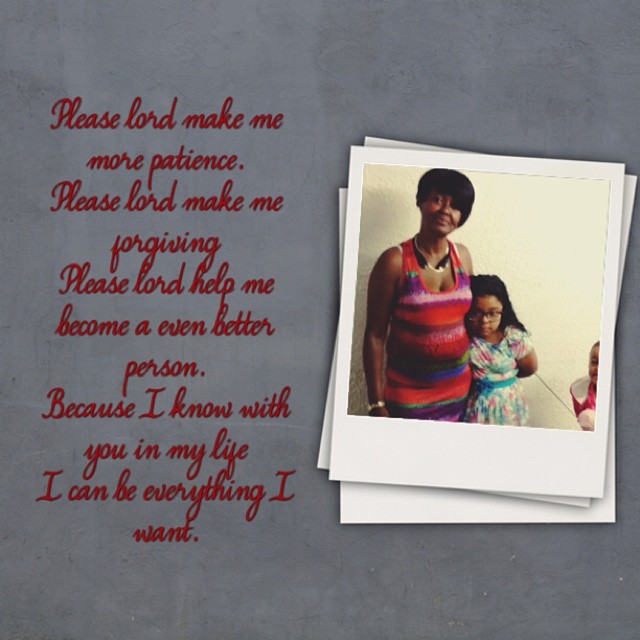This image features a heartfelt prayer on the left side, written in red cursive text on a grey background. The prayer reads, "Please Lord make me more patient. Please Lord make me more forgiving. Please Lord help me become an even better person because I know with you in my life I can be everything I want."

On the right side, a stack of Polaroid photos is depicted, with the top photo prominently showing a black woman and her two children standing in front of a plain wall. The woman, who appears pregnant, has long black hair and wears a sleeveless, horizontally-striped dress in shades of purple, red, green, and blue. She accessorizes with a black and white necklace. The little girl in the middle has long curly hair and eyeglasses. She wears a floral dress with a turquoise belt around the waist. To the right is another child, either a young boy or girl, partially visible and smiling, wearing a red and white shirt or dress. These elements collectively create a touching and colorful family portrayal alongside the pious text.